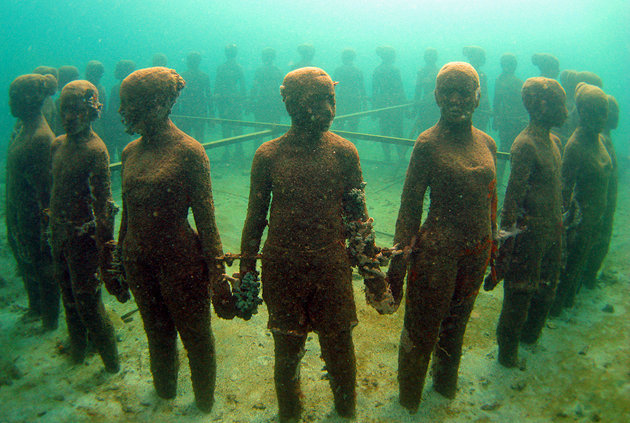This color underwater photograph captures a hauntingly beautiful scene of approximately 20 to 30 human-like stone sculptures arranged in a 360-degree circular formation with their backs to the center. The statues, a mix of male and female figures, appear to have been underwater for an extended period, as evidenced by their rust-colored, oxidized surfaces and thick coatings of crustaceans. The murky greenish-blue water bathes the scene in an eerie light, and sunlight penetrates the surface, casting a golden glow on the ocean floor where the statues stand. Circular rope or bands connect each figure, with crisscross bars providing support, ensuring they remain upright. The feet of the statues are buried in the sand, and they all face outward, creating a striking and mysterious underwater tableau.